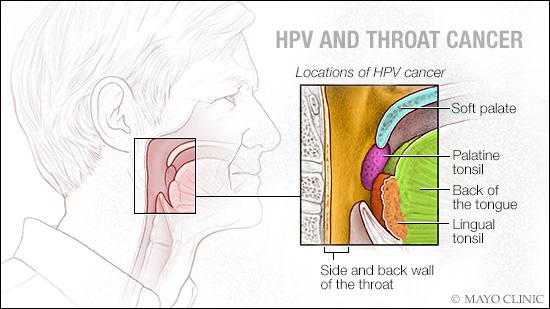This landscape-oriented, color illustration from the Mayo Clinic serves as an awareness-raising image for HPV and throat cancer. The background is white with "HPV and Throat Cancer" written at the top in gray font, and "Locations of HPV Cancer" underneath in black font. The bottom right corner features the Mayo Clinic logo in gray.

On the left side of the image, there is a detailed pencil sketch of an elderly man’s head in profile. His hair and skin are depicted in white, with a focus on his throat. Overlaid on this sketch is a highlighted area in light pink colored pencil, indicating the parts of his throat susceptible to HPV-related cancer.

The right side of the image contains the only color elements, featuring a close-up, hand-drawn depiction of the inside of a human throat in colored pencil. This illustration includes labeled arrows pointing to various parts of the throat: the soft palate, palatine tonsil, back of the tongue, lingual tonsil, and the side and back wall of the throat. This informative diagram effectively guides viewers to the locations where HPV-related throat cancer can develop, making it a comprehensive educational tool.